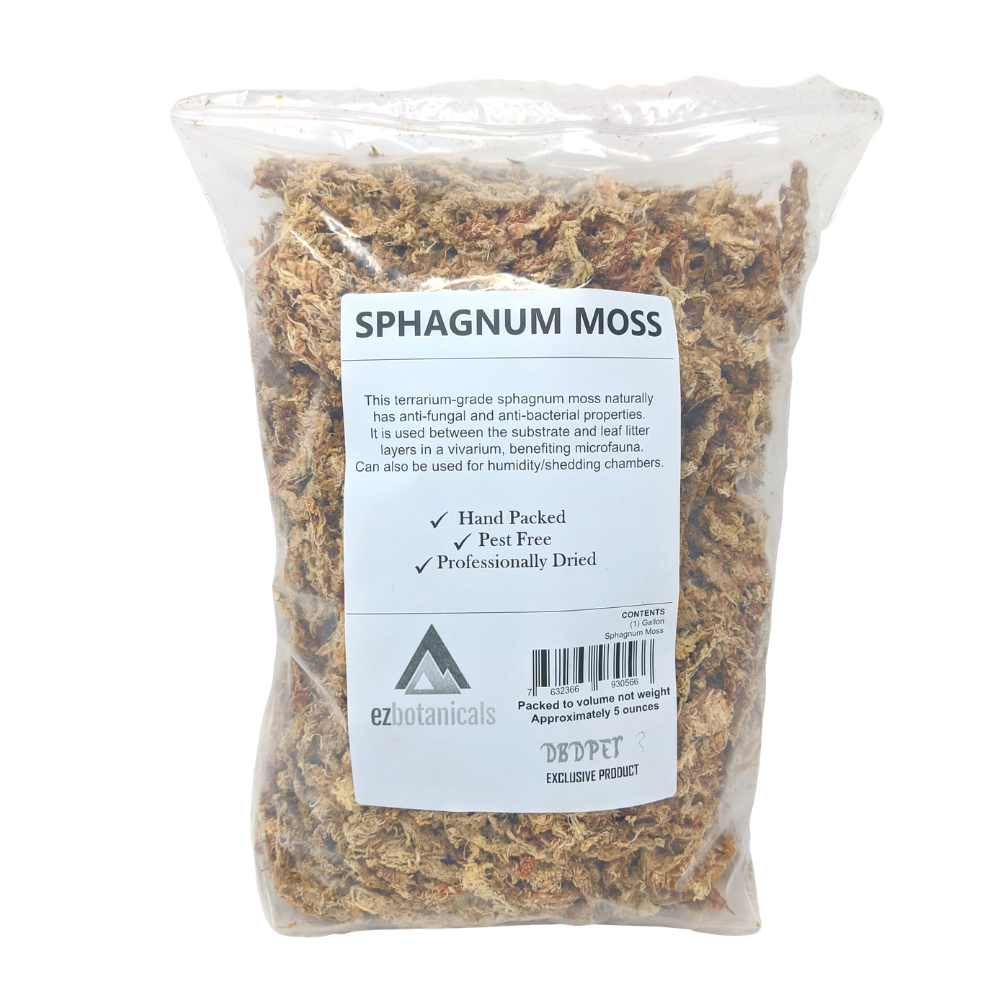This image features a clear, sealed plastic bag containing earthy, brownish-tan sphagnum moss with slight hints of green. The bag has a white label at the top with "S-P-H-A-G-N-U-M Moss" prominently displayed in black font. Below this, the label provides details about the moss, including its terrarium grade and natural antifungal and antibacterial properties. It mentions its use in vivariums, benefiting microfauna, and also as a component for humidity shedding chambers. Three check marks highlight that the moss is hand-packed, pest-free, and professionally dried. Below this information is another black line, followed by an emblem for the company Easy Botanicals on the left and a barcode with weight information on the right. The entire background of the image is completely white, which makes the details on the label and the contents of the package stand out clearly.